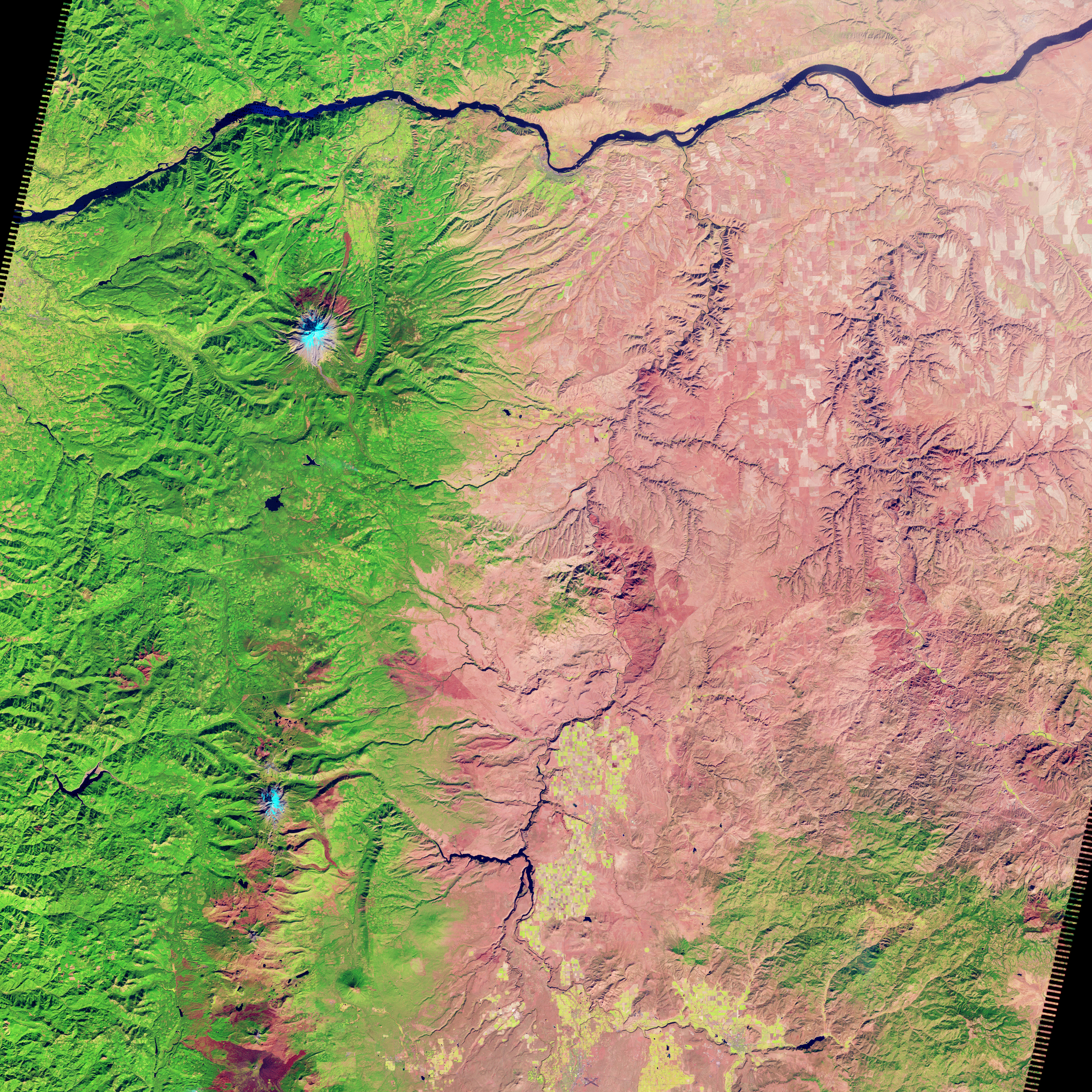This satellite image showcases a rugged landscape predominantly characterized by hard red clay terrain interspersed with verdant areas and small bodies of water. The left-hand side features green expanses, including low-lying foothills or depressions and two small lakes. A dark blue river or tributary system slices across the top portion of the image, descending toward the left. There are noticeable manipulations at the corners of the map, particularly the top left and bottom right. The barren red clay area, rich with cracks and fissures, suggests possible groundwater seepages forming minor waterways at the bottom. The right side comprises a mix of pink and white areas, signifying lower terrain among finer river networks leading into the larger river above. This detailed topographic overview, set against a dark black background, also includes some rugged ridges and sporadic white patches indicative of potential snow-capped peaks or sandy lowlands, adding to the terrain's varied texture. Overall, the image depicts a landscape of stark contrasts, with splotches of green and brown, ridges, valleys, and craters, providing a complex yet comprehensive aerial view of the area.